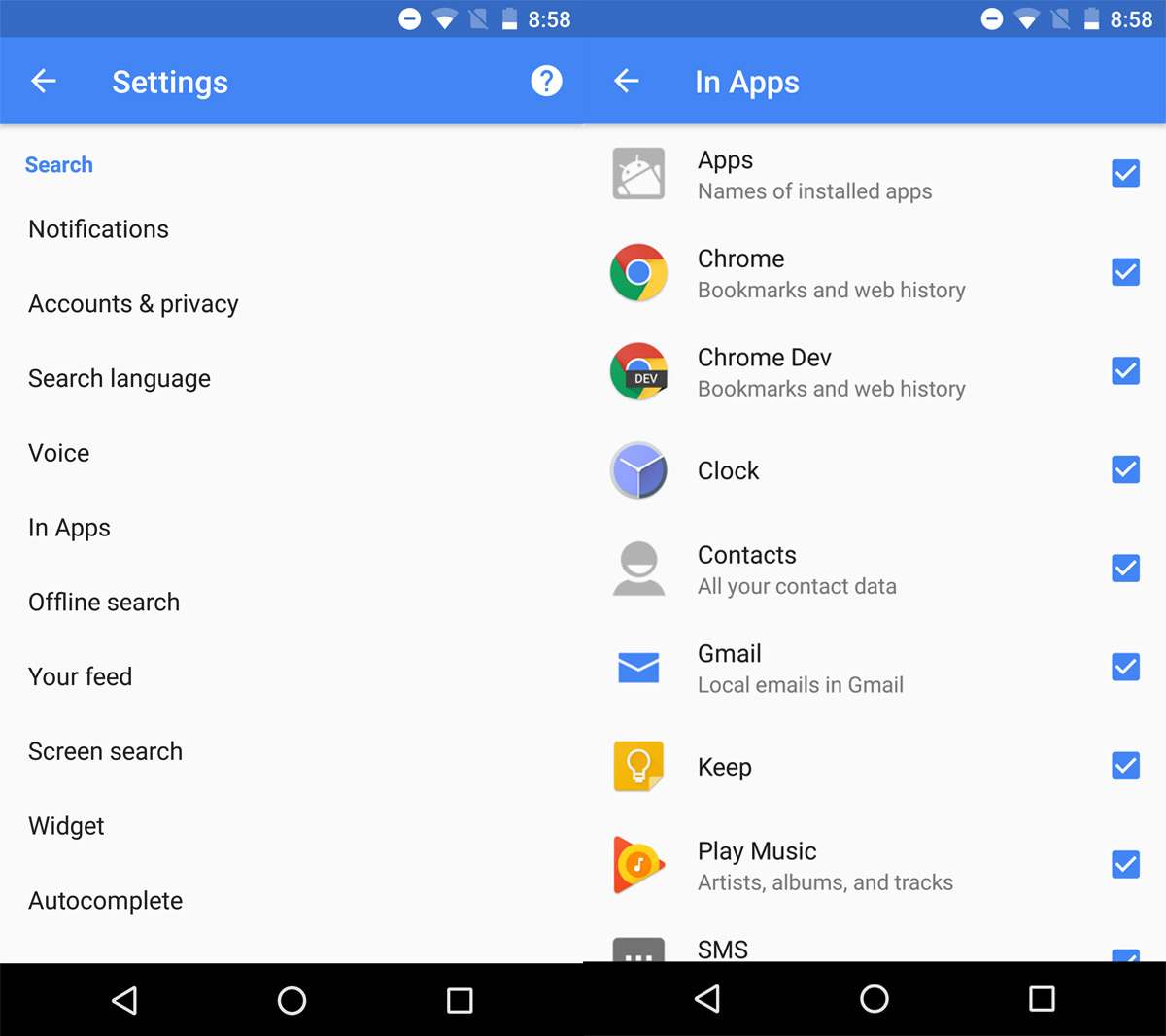This image consists of two edited mobile screenshots positioned side-by-side, displaying app settings and in-app settings respectively. Both screenshots feature a blue banner at the top. 

On the left, the banner has "Settings" written in large white letters with a left-pointing arrow beside it. Directly below the banner is a search bar followed by a vertical list of options in black text. The listed options include:
1. Notifications
2. Account
3. Private accounts and privacy
4. Search
5. Language
6. Voice
7. In-apps
8. Offline research
9. Your feed
10. Screen search widget
11. Autocomplete

On the right, the banner reads "In-apps" with a left-pointing arrow at the top of the screenshot. Below the banner, there is a vertical list of Google apps, each with a checkbox on the right side. The listed apps include:
1. Apps (with an Android icon beside it) - checked
2. Chrome - checked
3. Chrome Dev - checked
4. Clock - checked
5. Contacts - checked
6. Gmail - checked
7. Keep - checked
8. Play Music - checked
9. SMS - checked